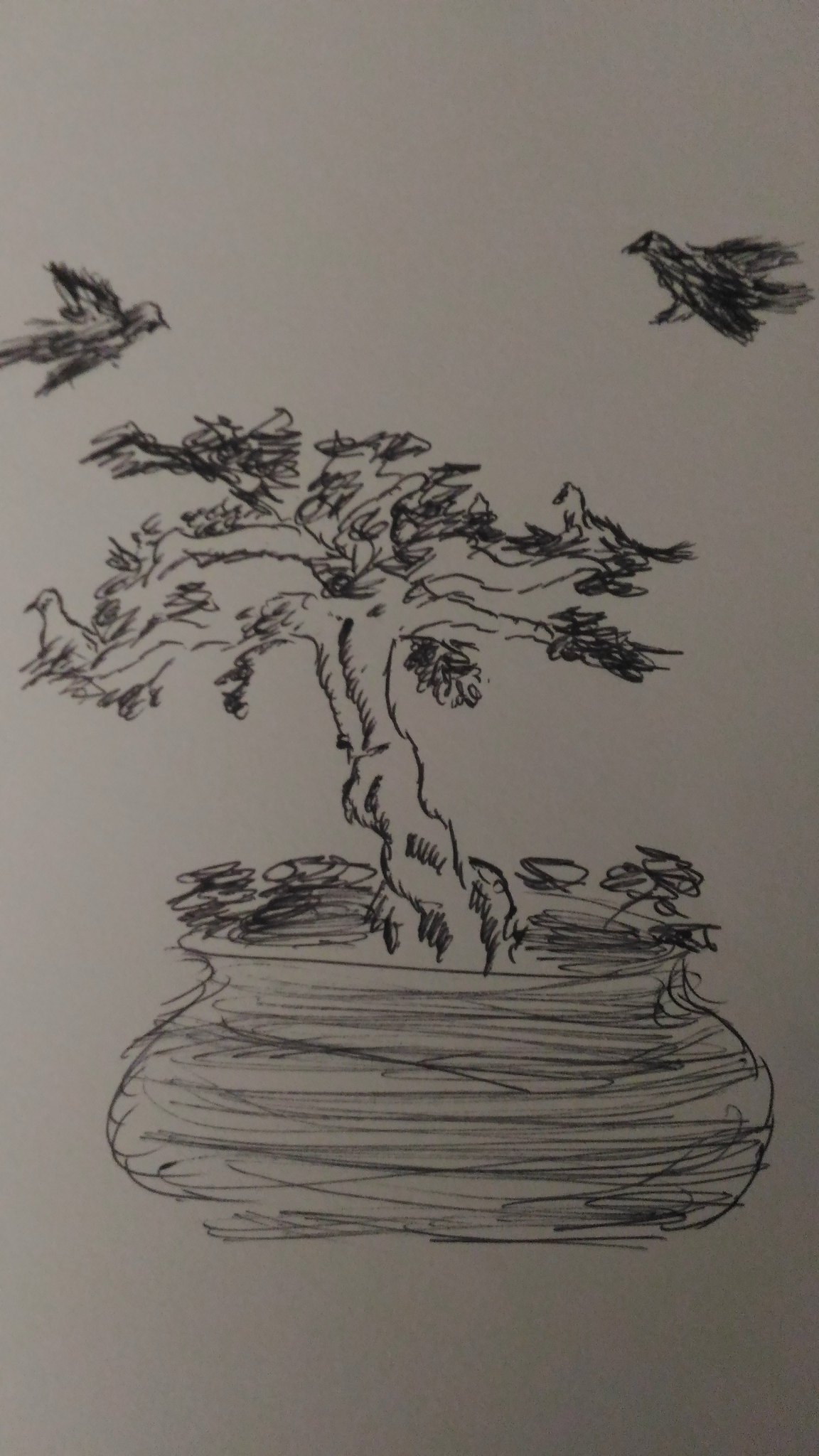The image is a vertical, slim pencil sketch on a piece of paper with a white background. It features a bonsai tree growing out of a pot, which appears to be sketched using black ink with multiple shadings and negative space. The pot itself is detailed with numerous small lines, giving it a textured appearance, and it appears either hollow or filled with soil. The bonsai tree, depicted with scratch lines and proper shading, has branches adorned with leaves and intricate details representing knots and twists. 

Several birds are part of the composition: two birds are perched on branches, one on a far-left branch and another on a far-right branch. Additionally, a bird is seen taking flight from a middle branch. Two more birds are flying above the tree, one in the top-left corner and another in the top-right corner of the image. The birds are detailed, with shading that suggests the structure of their feathers. Interestingly, while most of the birds appear dark or singular in color, the ones resting on the tree appear white. The overall sketch, though scribbly and seemingly quick, captures the essence of a bonsai tree and its avian visitors with remarkable detail.